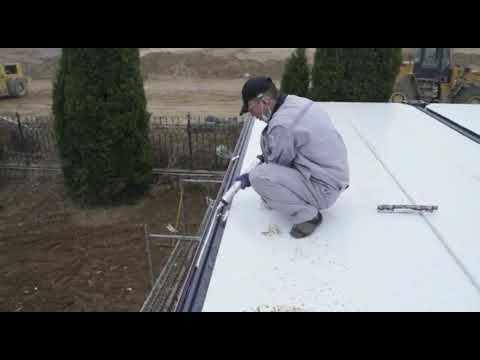The image depicts a young man, approximately in his 20s, engaged in repair work on a white, flat roof, possibly of a building. The photo appears pixelated and slightly blurry, suggesting it may be a screen grab from a video. The man is dressed in a light gray jumpsuit with long sleeves and pants, and he wears a black baseball cap. Around his chin, there's a safety mask, not covering his mouth or nose, and he appears to also have glasses.

In the photo, he is squatting with his hands extended between his legs, holding a caulking gun to apply white caulk to the edges of the gutter, sealing them. The ground below, which is visible, is a mix of browning grass and dried-out areas, indicating a late fall or winter setting. Evergreen trees and meticulously trimmed shrubbery can be seen in the background, along with construction equipment and yellow machinery further in the distance. There are also hills visible in the far background, adding depth to the setting.